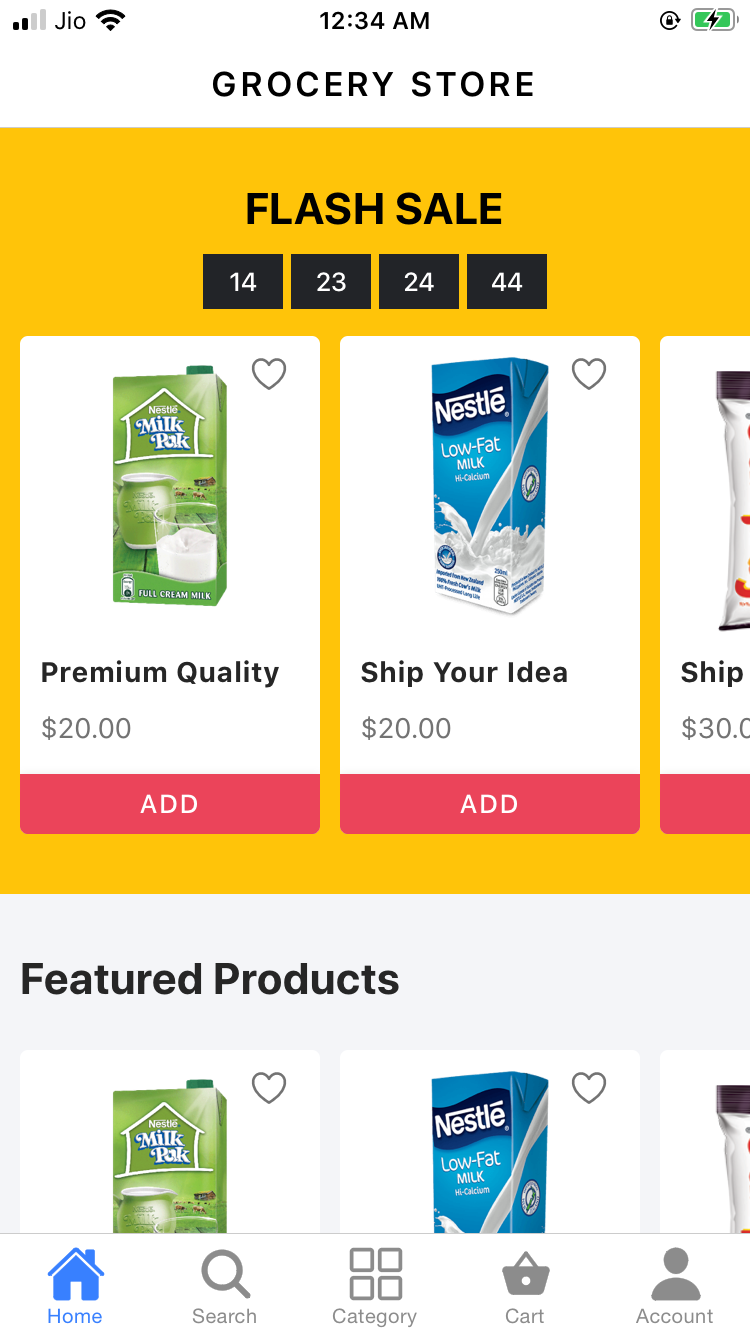A screenshot from an iPhone displaying a grocery shopping app. The iPhone shows two out of four bars of cellular service with "Geo" as the carrier, full Wi-Fi, and it is 12:34 AM with the phone on charge, almost at full battery. At the top of the app, the header reads "Grocery Store" in bold black text on a white background. A prominent yellow box with "Flash Sale" written in black catches the eye. The countdown timer below reads 14: 23: 24: 44.

In the Flash Sale section, several featured items are displayed. On the left, a "Premium Quality Milk Pack" is priced at $20 with a red "Add" button beside it. To the right, "Nestle Low Fat Milk" is available for the same price, with options to add it to the cart or mark it with a heart icon in the top right corner. Another item is partly cut off on the right side of the screen.

Below this section, under a light gray background labeled "Featured Products" in black font, the same Flash Sale products are displayed again, but only their tops are visible due to the bottom navigation menu obstructing the full view.

The bottom menu includes five icons from left to right: Home (a blue house), Search (a magnifying glass), Category (four squares), Cart (a shopping cart), and Account (a person). The Home icon is highlighted in blue, indicating the active tab, while the others are in light gray.